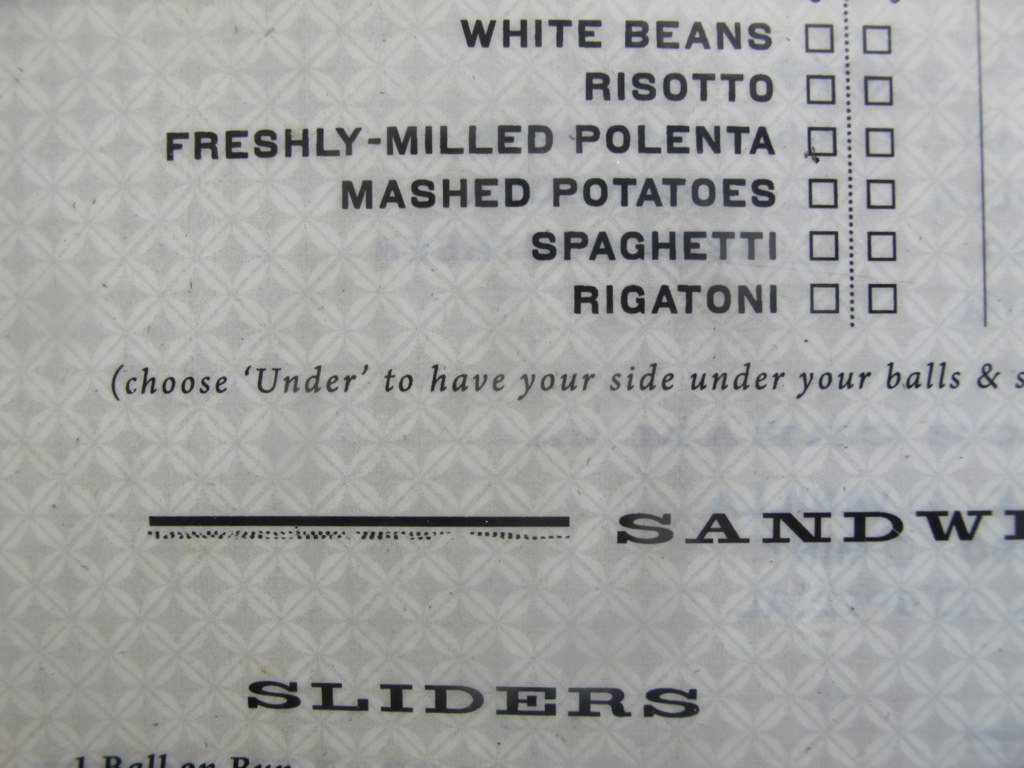This photograph captures a detailed view of a menu layout. The background features a gray and white houndstooth pattern, giving it a contemporary and stylish appearance. The menu has two sections distinguished by black letters and includes checkboxes for each option. 

One section lists side dishes with accompanying empty checkboxes:
1. White Beans
2. Risotto
3. Freshly Milled Polenta
4. Mashed Potatoes
5. Spaghetti
6. Rigatoni 

Next to each side dish name, there's a dotted line followed by another checkbox and a solid line. A note in parentheses reads, "Choose under to have your side under your balls," implying a customizable order method.

The menu also features bold black headings, one of which reads "Sandwiches" with a smaller subheading directly below, also in black letters, spelling out "Sandwiches" again as "S-A-N-D-W-I-C-H-E-S". Another bold heading spells "Sliders" as "S-L-I-D-E-R-S", clearly separating sections of the menu.

This detailed and organized design helps patrons easily select their desired meal options.